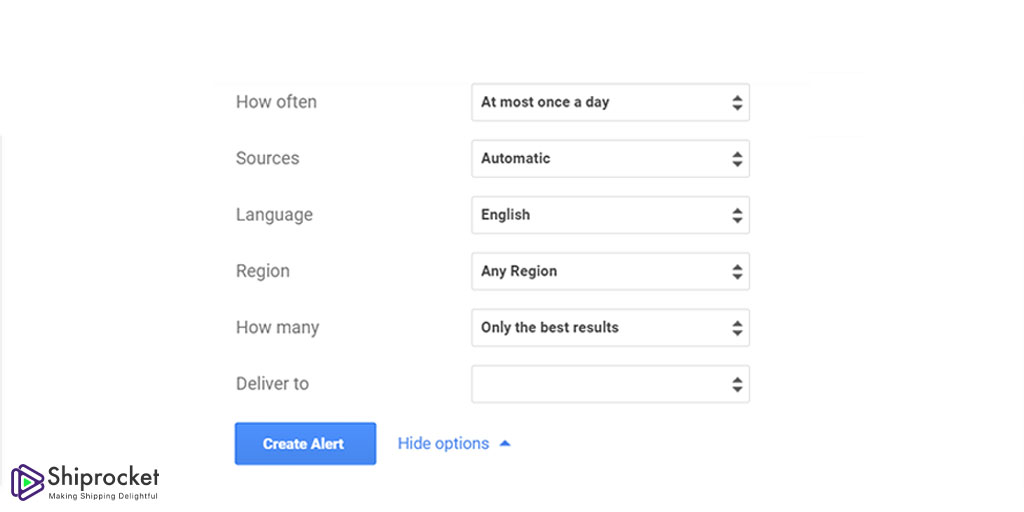The image is from Shiprocket, prominently featuring the brand's logo and slogan in the bottom left-hand corner. "Shiprocket" is written in black font with a capital 'S,' followed by the slogan "Making Shipping Delightful" in a smaller black font. To the left of the text is the Shiprocket logo, which consists of three bars that form an abstract 'S' shape. The top two bars are vertical and lean at their tips, while the bottom bar lies horizontally at an angle, touching the bottoms of the top two bars. The entire logo is slightly tilted to the left.

In the center of the image, there are several form fields and selection options. The "How Often" field indicates that the choice "At most once a day" is selected. Under "Sources," "Automatic" is selected, while "Language" is set to English. The "Region" field shows "Any Region" as the selected option. The "How Many" category has "Only The Best Results" chosen. At the bottom of this selection area is a prominent "Create Alert" button.